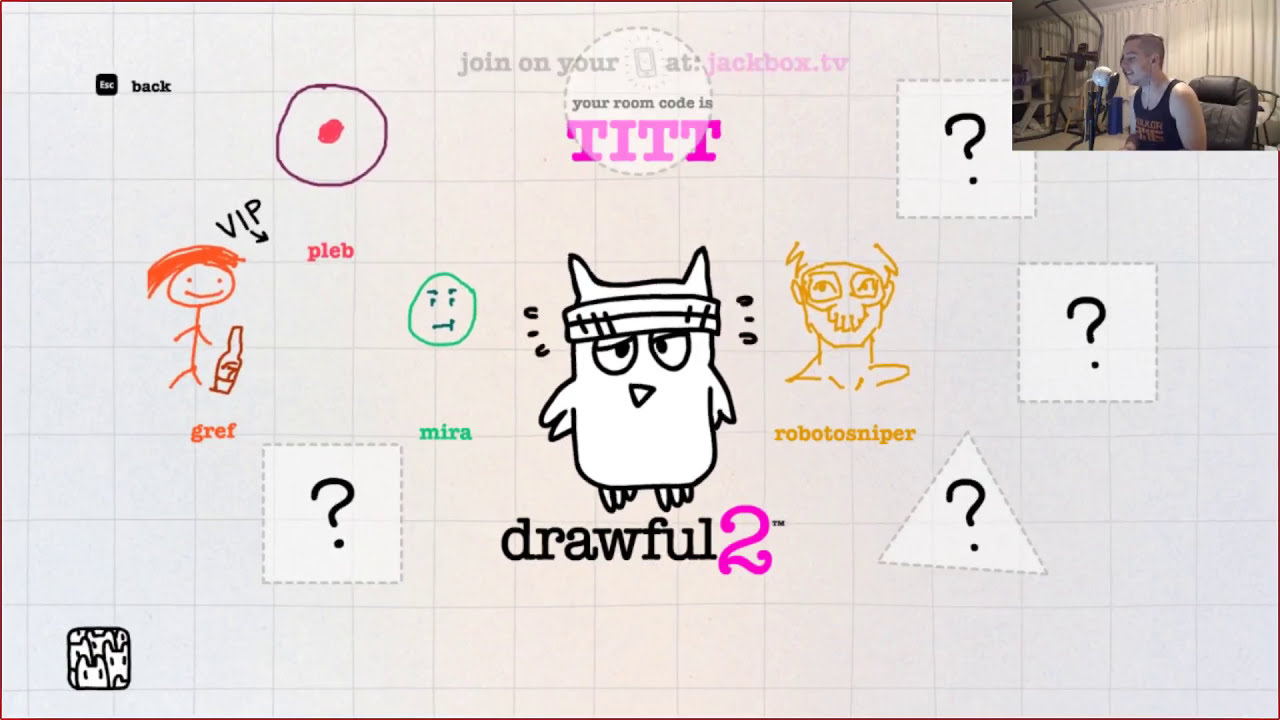The image depicts a rectangular screenshot from a live-streamed session of the game "Drawful 2." The screenshot is surrounded by a thin red pinstripe border and features a light gray background with grid lines. Prominently in the center, the game's logo, "Drawful 2," is displayed beneath a doodle of a white owl with two little horns and a headband. The text "Drawful" is in black, and "2" is in pink. Above this, there's game-related text that reads, "Join on your cell phone at jackbox.tv," followed by "Your room code is TITT," enclosed within a dotted circle.

The scene also includes various hand-drawn doodles contributed by players, each labeled with a username: "Roboto Sniper" next to a human head with a skull cap, "Mira" next to a green circle with a face inside, "Gref" below an orange stick figure reaching for a bottle, and "Pleb" associated with a small arrow. Additionally, several squares and triangles with question marks indicate slots for more players. 

In the upper left corner, there is a black button labeled "ESC" for escape, and beside it, the word "Back" in black letters. The upper right corner features an inset of a male streamer smiling while sitting in a black chair. The streamer, who is Caucasian and wearing a black tank top with gold print, is possibly engaged with the game, adding a lively element to the scene. This comprehensive view integrates gameplay instructions, the active participation of users, and the engaging environment of a live stream.